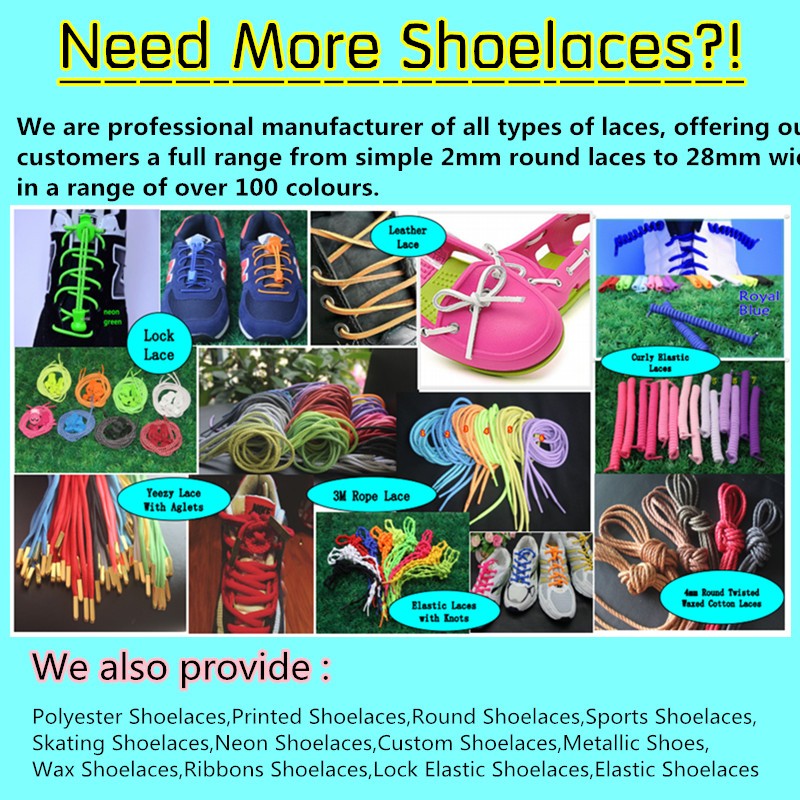This square advertisement features a vibrant blue background that immediately catches the eye. At the top, bold yellow letters underline the question, "Need more shoelaces?" Below this, a central arrangement of various images displays an assortment of shoes and shoelaces showcasing diverse colors and styles. The main text in the center proudly states, "We are a professional manufacturer of all types of laces, offering customers a full range from simple 2mm round laces to 28mm wide, available in over 100 colors." Several images highlight the colorful options, including light blue, yellow, black, lime green, orange, navy blue, pink, and purple laces. Additional text under these images elaborates on their offerings in bold red letters: "We also provide polyester, printed, round, sport, skating, neon, custom, metallic, wax, ribbon, lock elastic, and elastic shoelaces." The varied positioning of the shoelaces and shoes within the ad gives it a dynamic, presentation-like feel, effectively demonstrating the extensive variety available from this professional shoelace manufacturer.